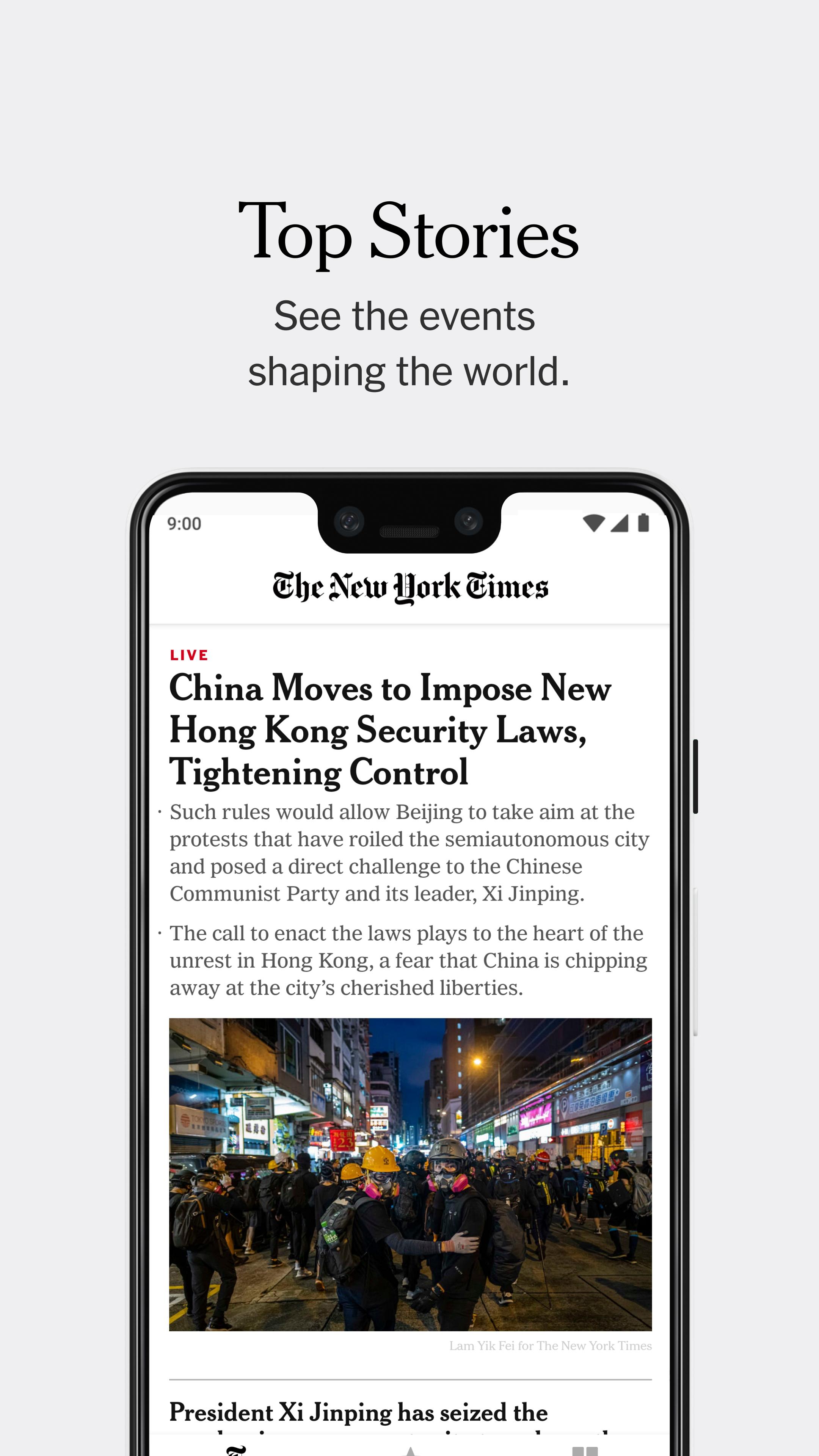The image features a sleek gray background with prominent, large, bold black text at the top that reads "Top Stories: See the Events Shaping the World." Below this header is a smartphone screen illustration. 

In the top left corner of the phone display, the time is shown as 9:00, while the top right corner features standard status icons for battery life, Wi-Fi, and cellular signal. The screen showcases The New York Times app interface. 

A horizontal line spans the width of the display under the app title, with the word "LIVE" written in red on the left. Just beneath this, a headline in black text reads, "China Moves to Impose New Hong Kong Security Laws, Tightening Control." 

Smaller text below the headline elaborates: "Such rules would allow Beijing to take aim at the protests that have roiled the semi-autonomous city and pose a direct challenge to the Chinese Communist Party and its leader, Xi Jinping. The call to enact the law plays to the heart of the unrest in Hong Kong, a fear that China is chipping away at the city's cherished liberties."

An image is shown beneath the text, depicting a bustling protest scene with numerous people in the street surrounded by vibrant neon lights illuminating the left and right sides of the crowd.